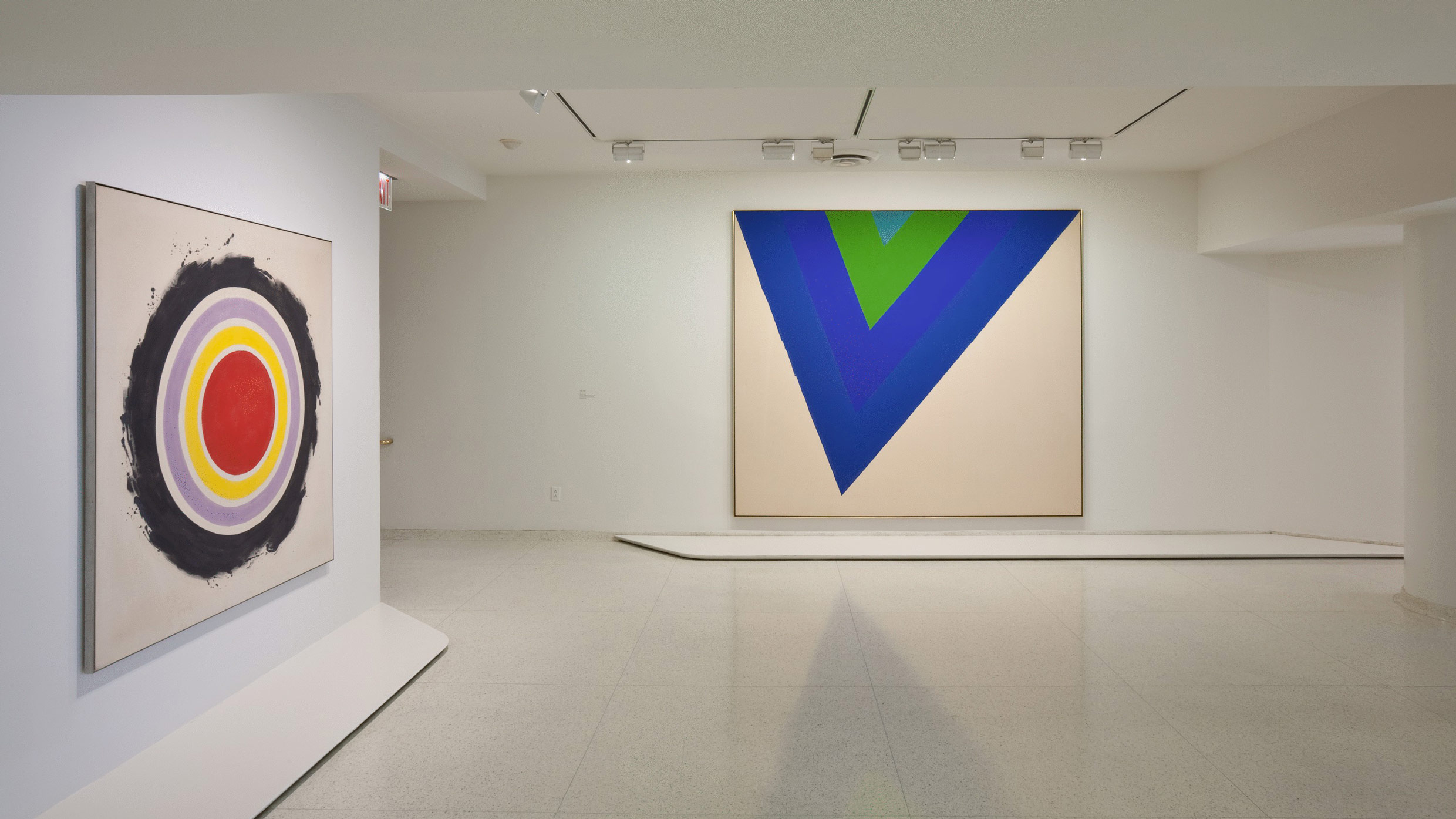The image captures the interior of a stark, sparse art gallery with white walls, ceiling, and a light-colored, white-paneled floor. In the gallery space, irregularly placed walls create a somewhat segmented appearance. Two large abstract paintings are prominently displayed. On the left wall, a painting features a series of concentric circles resembling a bullseye: a central red circle, followed by a yellow ring, a purple ring, and a roughly painted black ring, all on an otherwise white canvas. The rear wall showcases a geometrically patterned painting with a white field. Dominating the canvas is a large blue triangle pointing downward, nearly reaching the bottom. Superimposed on this is a centered green triangle, and within that, a light blue triangle. The two paintings almost stretch from the floor to the ceiling, contributing to the minimalist aesthetic of the gallery.